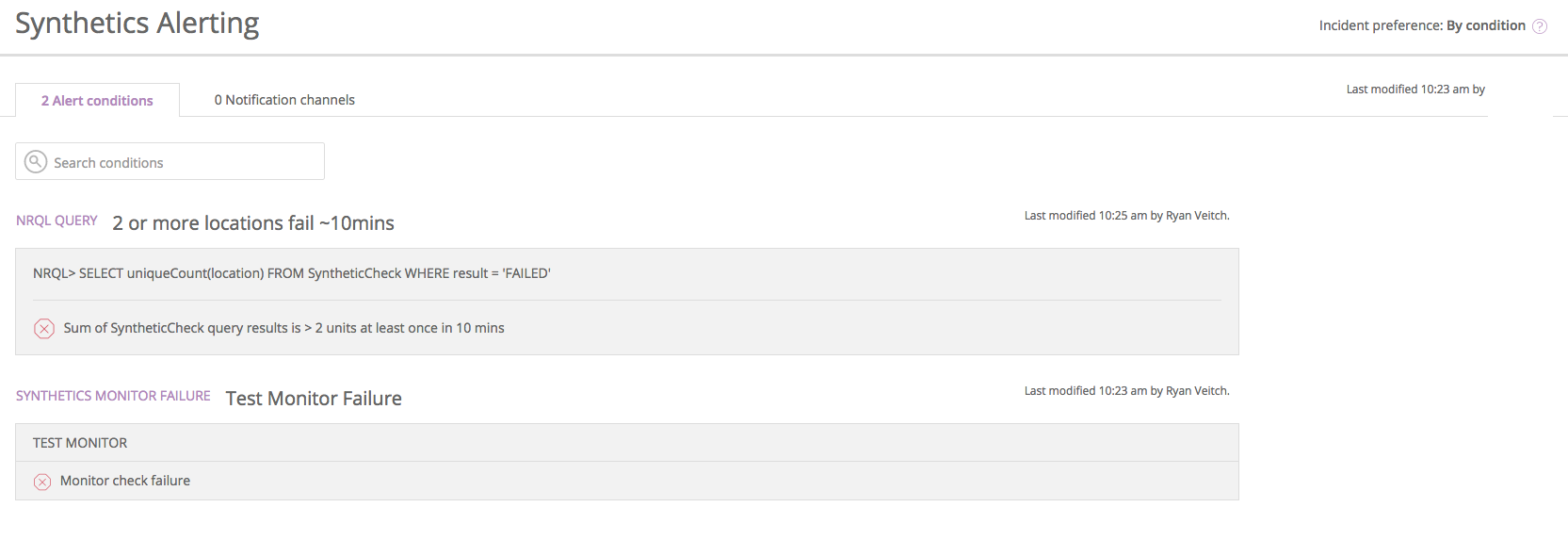The website showcased in the image has a minimalistic and somewhat monotonous design. In the upper left-hand corner, the title "Synthetics Alerting" is prominently displayed. Just below it, a gray navigation bar extends horizontally across the entire width of the page. Above this line, the text "Incident Preferences by Condition" is clearly written, with the note "Last Modified: 10:23 AM" right beside it.

Below the "Synthetics Alerting" header, there is a section marked by two alert conditions highlighted in purple, labeled "Notification Channels." A search box titled "Search Conditions" is present for filtering criteria. The section contains information about an NRQL query. This query appears to check if two or more locations fail or fall within a 10-minute window. 

A gray box beneath this displays the NRQL statement: "SELECT uniqueCount(core) FROM SyntheticCheck WHERE result = 'FAILED'". Adjacent to this, a red circle with a red X icon visually signifies an error or failure, indicating that some synthetic check query results failed at least once within the past 10 minutes.

Additionally, there is a section labeled "Synthetics Monitor Failure," which includes a subsection for "Test Monitor Failure." Contained within is a box titled "Test Monitor” with another red circle and red X icon, denoting a monitor check failure.

On the right side of the page, the modification timestamp appears again, stating "Last Modified: 10:23 AM by Ryan Welsh."